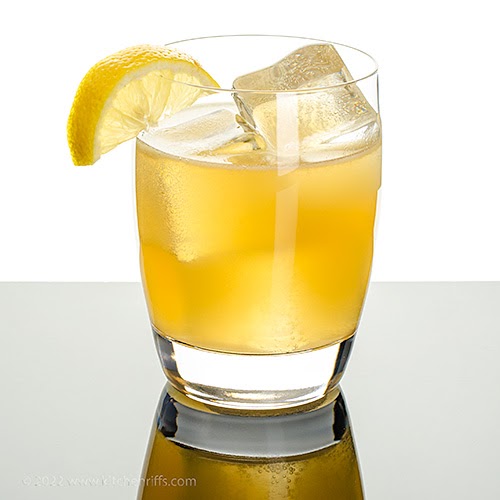This photograph captures a simple, yet striking image of a short, slightly rounded glass at the very center, resting on a mirrored, gray surface. The liquid inside the glass is a dark yellow, possibly lemonade, and condensation forms on the glass, suggesting its cold, refreshing nature. Two large ice cubes float within the drink, one peeking higher on the right. A small half-slice of lemon delicately adorns the rim, adding a touch of vibrancy. The pristine white background creates a clean, minimalist aesthetic, further highlighting the lemonade glass that is centrally and prominently featured. The reflection of the glass on the mirrored surface below adds depth to the composition, underscoring the simplicity and elegance of the visual. The text "2022 www.kitchenriffs.com" is faintly visible in the bottom left corner of the image.